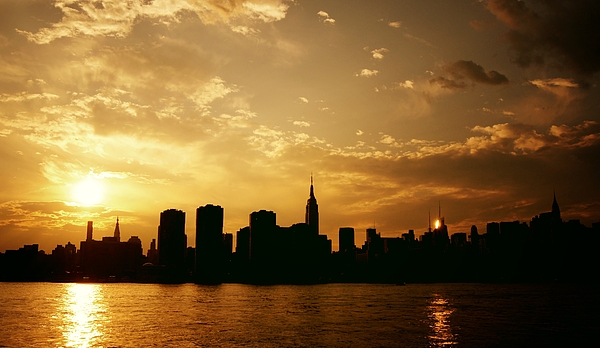The image captures an outdoor scene, likely during sunrise or sunset, highlighting a vibrant, orange-hued sky with variations of yellow radiating around the sun. Puffy white clouds, all tinged with shades of orange, dot the sky. In the foreground, several buildings of various shapes and sizes adorn the skyline—some wide, some thin, and some with tapered tops finishing in thin poles. The city's silhouette appears with brownish tones, and distinctive structures like steeples and high-rises stand out. Below the skyline, a calm body of water mirrors the glowing sun and the buildings, creating a serene, reflective surface amidst the overall darkened foreground, which transitions to a brighter left side as the sun ascends or descends.